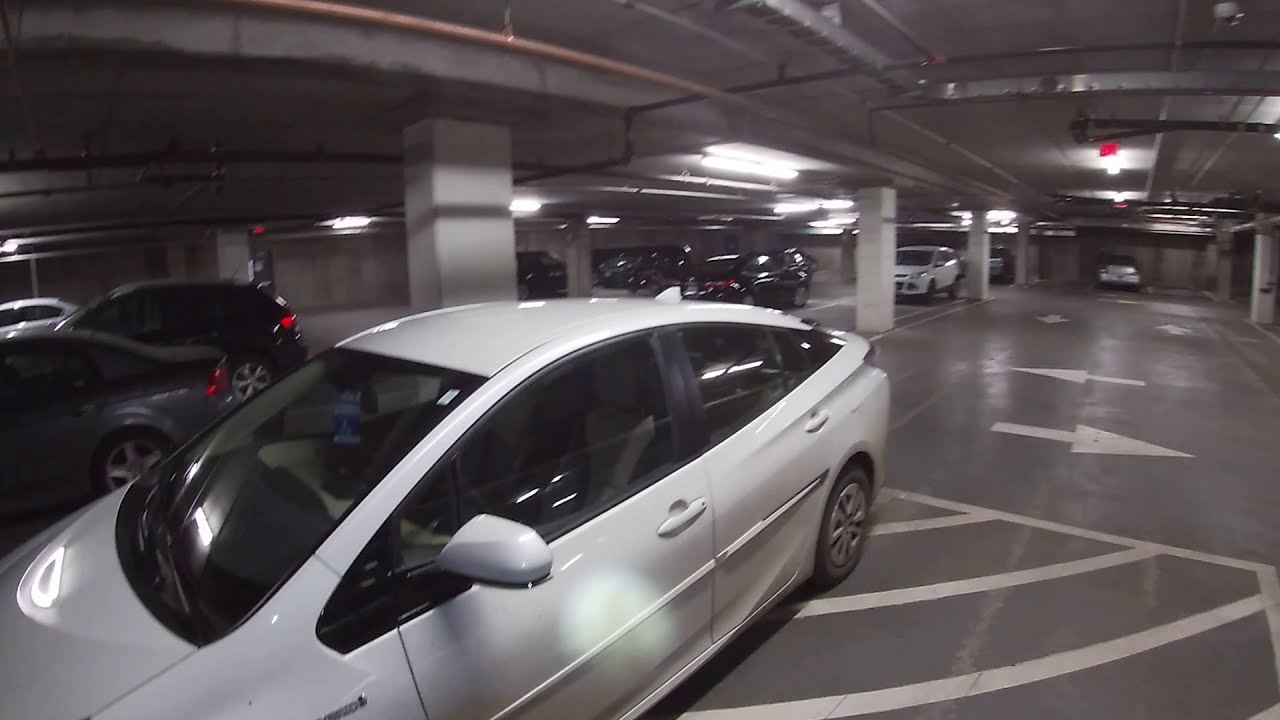The image depicts an indoor, multi-level parking garage in the U.S., characterized by a concrete structure with visible pillars and piping hanging from the ceiling. Fluorescent lights illuminate the space, casting a somewhat dim atmosphere. The floor is marked with directional arrows indicating ingress and egress, guiding vehicles in various directions. In the foreground, a white, four-door sedan with silver tire rims is prominently featured, positioned slightly off from the designated parking lines, suggesting it may be parked in a restricted area. The car's back end appears slightly smooshed, giving it an aerodynamic look. Behind it, several additional cars are parked in neat rows with clear parking lines. The garage is not overly crowded, housing approximately ten visible vehicles. Some sections of the floor have pedestrian walkways distinct from the parking spaces. No people are present in the scene, but an exit sign is noticeable among the various concrete features.